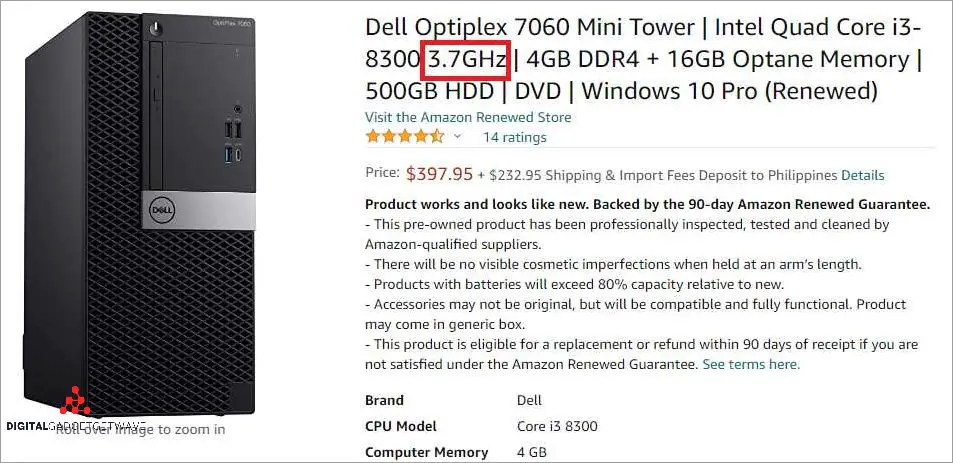This image displays a detailed Amazon listing for a Dell Optiplex 7060 Mini Tower computer. The listing highlights key specifications, including an Intel Quad Core i3-8300 processor clocked at 3.7 GHz, which is emphasized with a red annotation box. It features 4 GB of DDR4 RAM, 16 GB of Optane memory, a 500 GB hard drive, and a DVD drive. The system operates on Windows 10 Pro and is sold as a renewed product.

Beneath the product details, the listing indicates its affiliation with the Amazon Renewed Store, boasting a 4.5-star rating based on 14 customer reviews. The price is set at $397.95, with an additional shipping fee of $232 from the Philippines, accounting for the higher shipping cost. A "Renewed" label ensures that the product looks and functions like new, backed by a 90-day Amazon Renewed Guarantee. Bullet points outline that the item is pre-owned but has undergone professional inspection, testing, and cleaning, assuring no visible cosmetic imperfections from an arm's length distance.

On the left, the image of the Dell Optiplex 7060 Mini Tower is shown, featuring the black tower’s mesh front panel, a vertically oriented DVD drive, and multiple USB ports and additional connectors on the front panel. The brand is listed as Dell, with a CPU model of i3-8300 and 4 GB of computer memory.